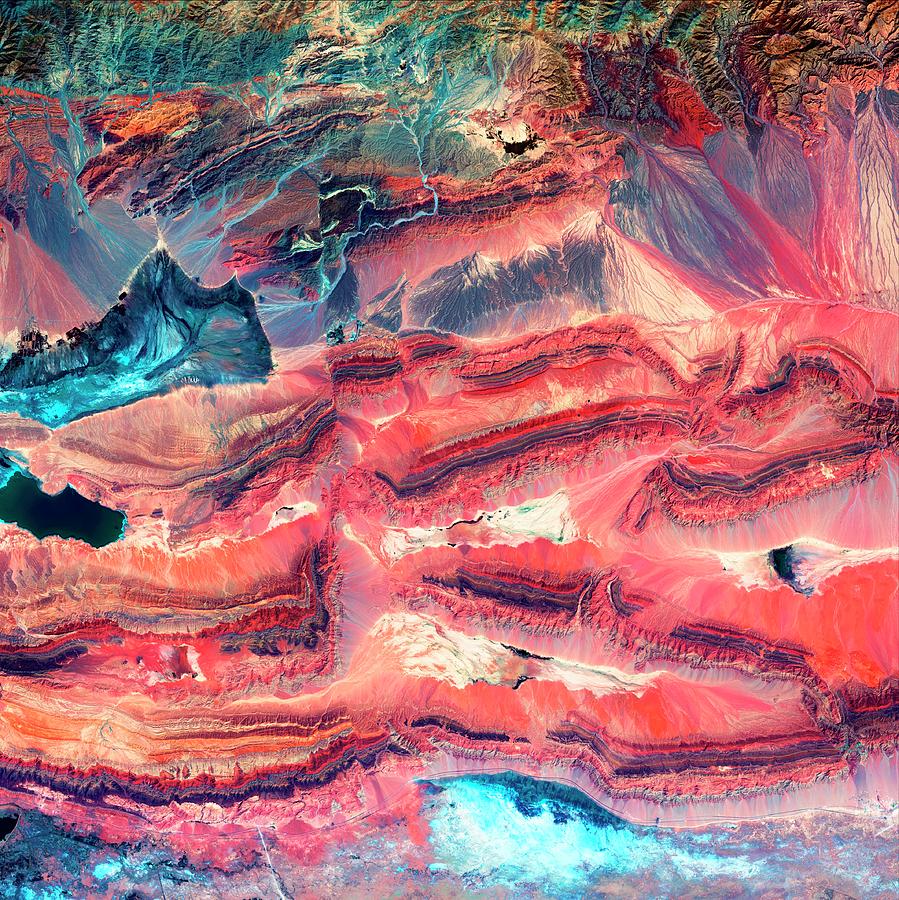The image intricately depicts a vivid, textured landscape resembling a geological cross-section, possibly of the earth's layers or a canyon-like structure. The uppermost section features a blend of brown and bluish-green, transitioning into a cascade of brown, orange, and reddish hues. Detailed blue lines suggest the presence of rivers or veins cutting through the cliff face. On the left, dark blue and cyan accents intersperse the orange-red layers, mirrored on the right with additional dark blue and red. This tier gives way to a mix of brown, dark blue splotches, and an enveloping orangish-red, creating a non-uniform, rugged texture akin to eroded mountainous terrain. The lower sections are characterized by a flat orangish-red expanse on the right and a convergence of red and blue tones at the base, culminating in a pure blue bottom right. The composition, with its vibrant palette of blues, purples, reds, oranges, and whites, mimics the intricate patterns found in nature, reminiscent of the Grand Canyon or a polished stone surface, infusing the scene with both natural beauty and artistic allure.